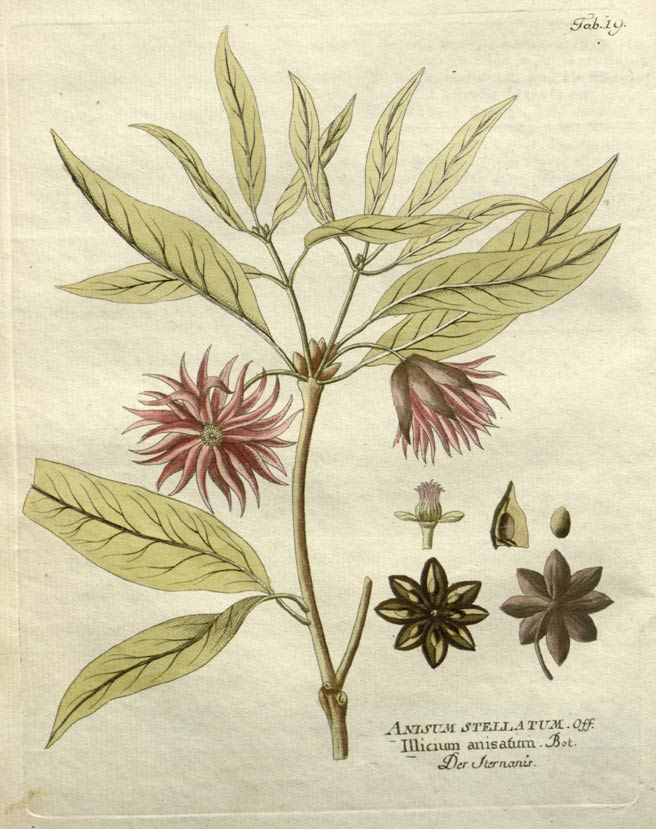The image appears to be a detailed botanical illustration on slightly sepia-toned paper. It depicts the stem of a plant that branches into smaller stems, each adorned with dull green leaves. At the top of the main stem, there are two prominent red flowers, one fully bloomed and the other just beginning to open. The petals of the flowers are intricate, resembling anemones with pointed, curvy shapes. Toward the bottom right of the illustration, beneath the canopy of leaves and flowers, are smaller images showcasing various parts of the plant, including flower buds, seeds, individual petals, and cross-sections of stems. The bottom part of the image contains some Latin text, likely identifying the plant, and in the top right corner, there is an inscription that reads "tab. it."